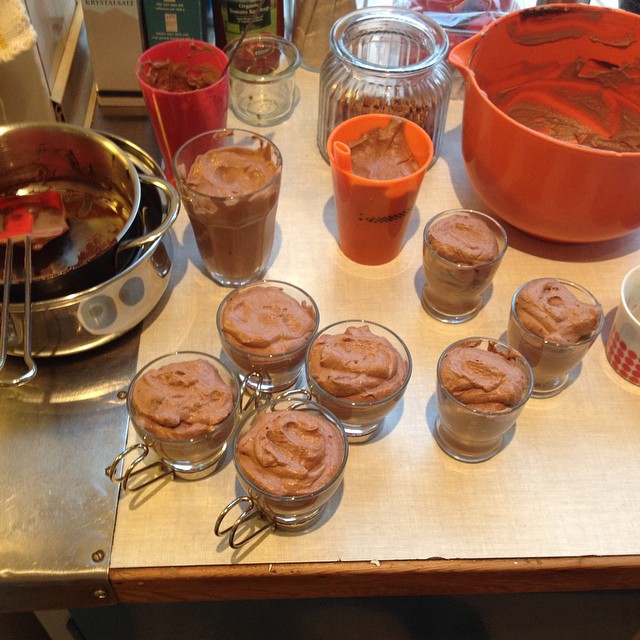In a bustling kitchen scene, there is a tabletop laden with various dessert preparations. A diverse assortment of glasses, cups, and jars are filled with a chocolatey batter, resting on a wooden surface that's partly covered with a white mat. On the far left, a double boiler made up of two silver pots stacked together holds remnants of chocolate, with a red spatula sticking out. In the middle foreground, four small jars with handles are filled to the brim with chocolate batter. Just behind them, a tall glass contains the same mix, and an orange plastic cup, resembling a sippy cup, is similarly filled. Also visible are a red cup and three shot glasses, each containing more of the chocolate mixture.

To the right, a large orange mixing bowl brims with a creamy, tan substance that looks like peanut butter. Nearby, there are additional containers: a pink cup, a glass jar, and an orange plastic cup, all filled with either the chocolate batter or the peanut butter-like mixture. Surrounding these are smaller glasses housed in metal holders, and additional utensils and props like a spoon sticking out from one of the cups. The countertop under the dessert array shows both wooden and stainless steel sections, suggesting a multi-functional kitchen workspace. In the background, hints of a home setting are visible, with light-colored cabinetry and glimpses of the floor.